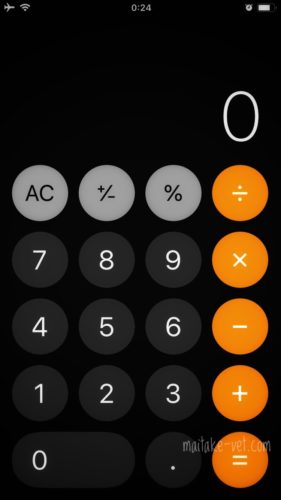This image showcases the Calculator app on an iPhone. At the top of the screen, the status bar is visible, displaying an airplane mode icon, indicating that the phone is in airplane mode. Additionally, the status bar shows the signal strength, phone carrier name, and battery icon, which is at 24%. Below the status bar and occupying the majority of the screen is the Calculator app, which is currently idle, displaying a zero since no calculations have been inputted yet.

The calculator interface starts with a row of three gray buttons, labeled "AC" for all clear, "+/-" for changing the sign of the number, and "%" for percentage calculations. Below this row are the number keys, arranged in a grid format with white text on black buttons. The numbers are laid out in a standard calculator layout: 7, 8, 9 in the top row; 4, 5, 6 in the second row; 1, 2, 3 in the third row; and '0' and a decimal point '.' at the bottom. 

To the right of the number keys are a column of orange buttons used for operations, each featuring a white mathematical symbol: division (÷) at the top, multiplication (×) below it, subtraction (−) next, and addition (+) at the bottom. The equal sign (=) button, also orange with white text, is situated at the bottom right corner, completing the setup of this intuitive and user-friendly interface.